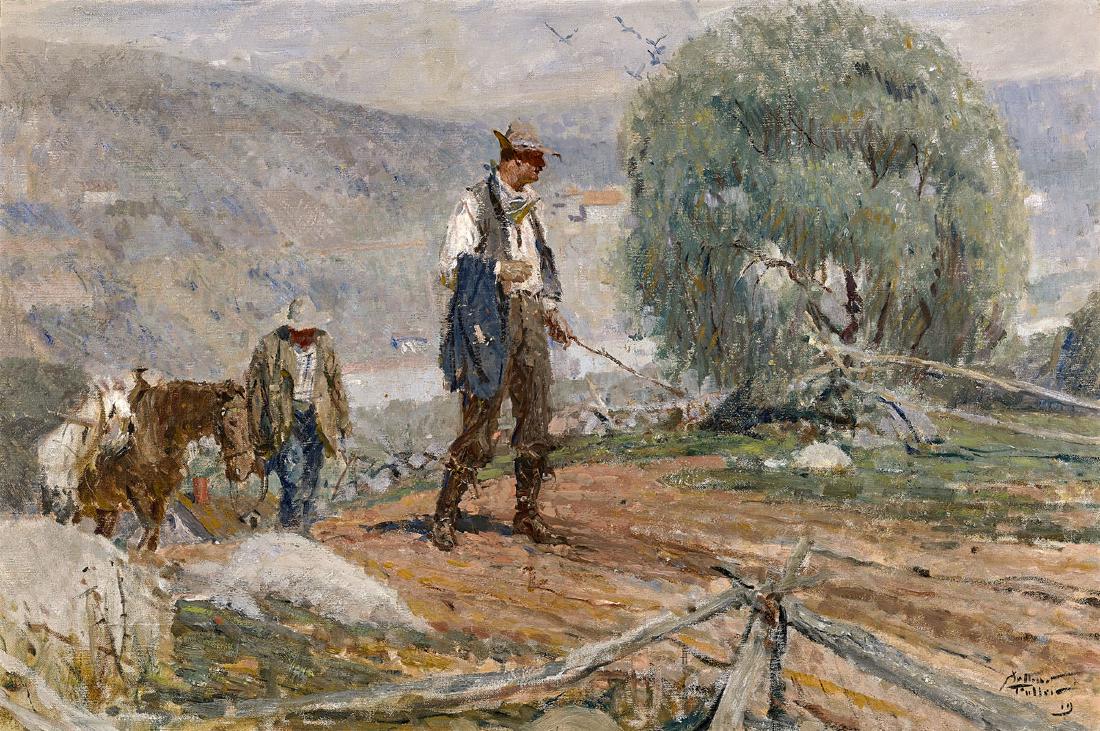This image is an old painting depicting a scene reminiscent of the American Old West, likely set in the 1800s. In the painting, two men are traversing a dirt road up a hill, with a picturesque backdrop of rolling hills, valleys, a few birds, and distant mountains. The scene features a palette of greens, tans, and whites, typical of an oil painting. 

The man in the foreground has a rugged appearance, wearing a brown cowboy hat with the front brim tilted down and the back flipped up. He is dressed in a long-sleeve white shirt, a vest, black trousers, and knee-high brown cowboy boots. He carries a stick in his left hand and drapes a blue jacket, possibly an old Army coat, across his arm. A small, illegible signature is visible in the bottom right corner of the painting.

Behind him is a second man, who has a light beige or tannish-green jacket, a white shirt, blue jeans, and a distinctive cowboy hat with flaps. He leads a horse outfitted with a saddle up the road. The path they walk on is framed by a weeping willow tree and low fencing, suggesting it might be there to contain livestock, such as sheep. The detailed portrayal captures the essence of frontier life and the rugged terrain of the countryside.